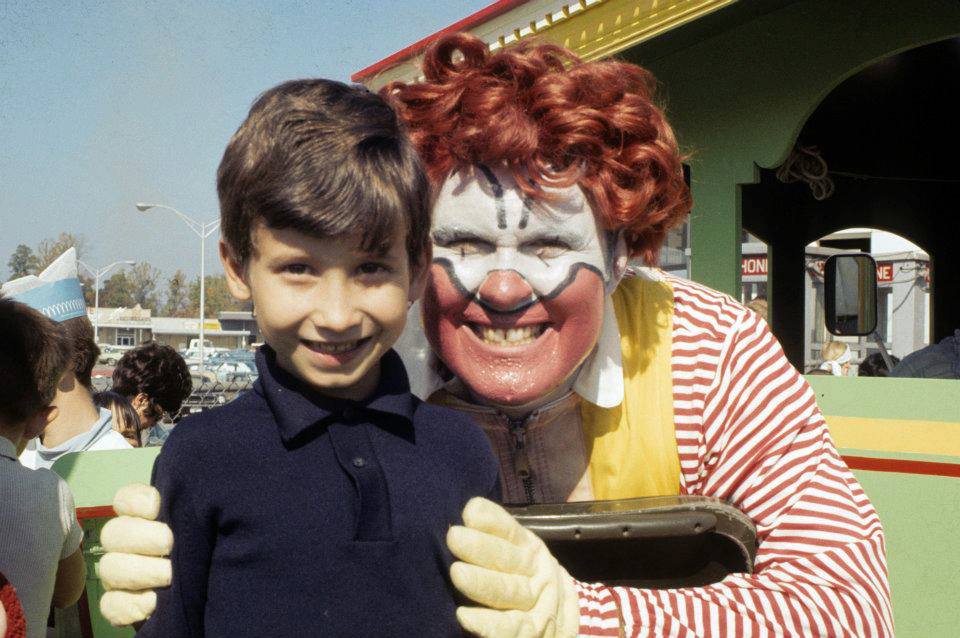In this color photograph, a young boy and a clown, who remarkably resembles Ronald McDonald, are posing happily outside a McDonald's restaurant. The boy, appearing to be around 5 to 8 years old, has short dark brown hair and wears a collared, long-sleeved navy shirt buttoned all the way up. Both he and the clown are smiling brightly. The clown, dressed in a red and white striped outfit with yellow accents, sports a bright red wig and white face makeup with bold red and black details, including black outlines on his cheeks. Yellow gloves complete his outfit. Behind them, the scene reveals a green building with yellow and red trim, indicative of an older photograph due to the film-like quality and the fabric hat of a man standing in the background, who is wearing a chef's hat. Also visible are a few cars and shopping carts in a large parking lot, suggesting they are in front of a McDonald's location that is part of a strip mall. Streetlights and cloudless skies further add to the atmospheric details of this nostalgic image.